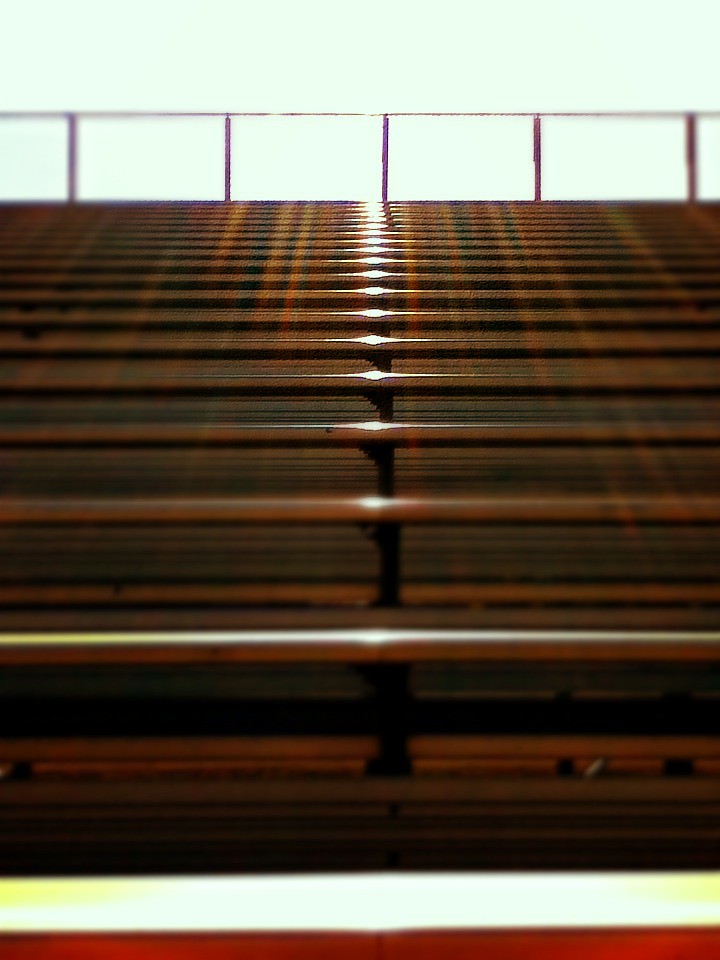Description of an image showing empty outdoor bleachers:

Amidst the stark, white sky, the sun beats down on a set of empty bleachers, casting a radiant glow that illuminates their bronze-brown surface. The bleachers, arranged in a successive, tiered fashion, stretch into the distance, with a railing crowning the top row. The sun's intense light creates a play of shadows that emphasizes the wooden texture of the bleachers, though the material might be an illusion from the harsh sunlight. The entire scene, devoid of any people or text, suggests a setting in an outdoor venue like a football field or an amphitheater. The midday sun underscores the stillness and emptiness of the scene, highlighting the solitary and serene nature of the moment captured.